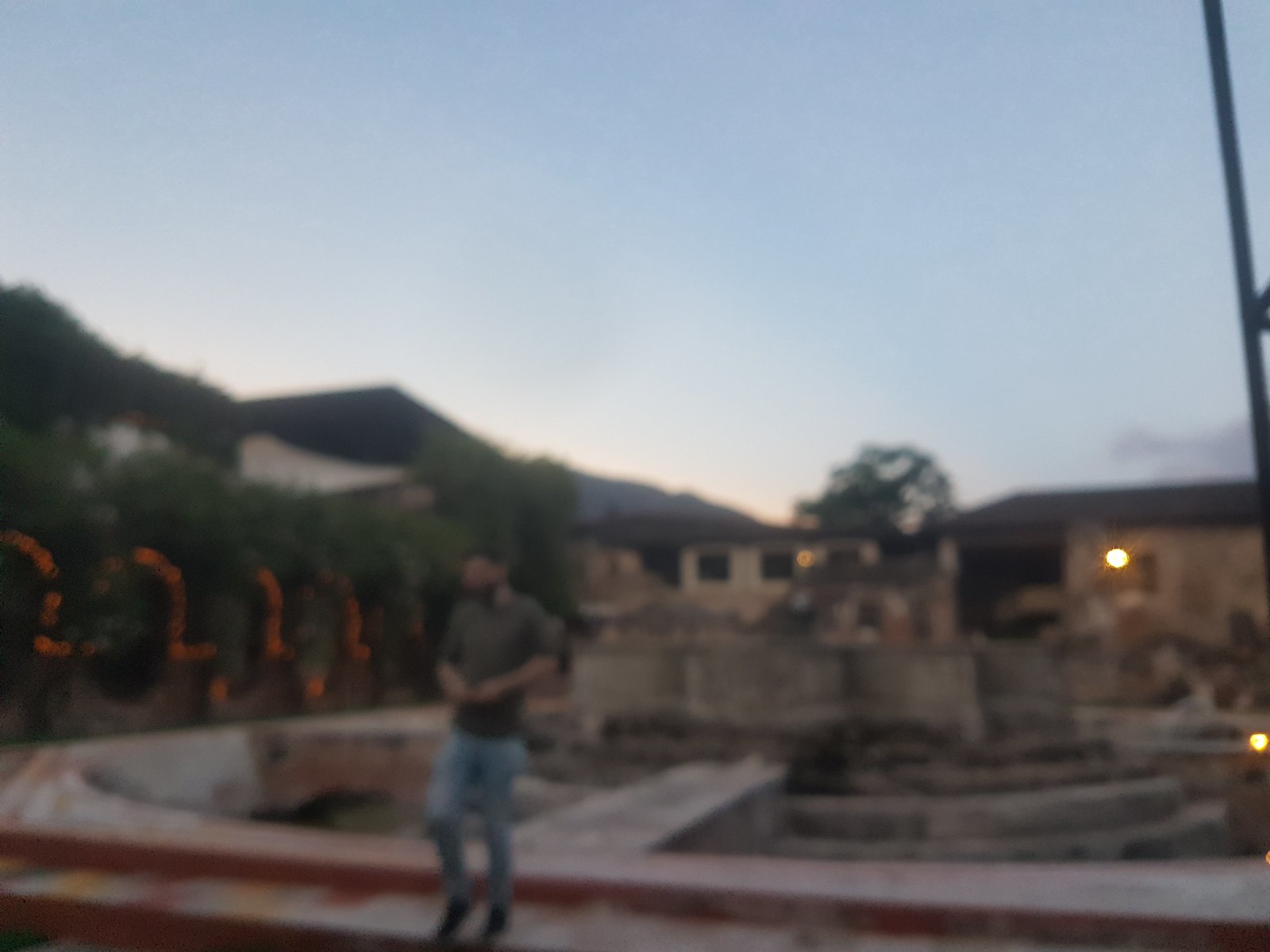In the foreground of this photograph, a man stands with his arms folded, wearing blue jeans and a dark shirt. Although his features are indistinct due to the blurriness of the image, his posture and attire are clear. Behind him, a building that appears to be a home is softly illuminated, with its lights casting a warm glow through the windows. The exterior details of the house, including windows and a walkway, are visible despite the overall blur. The sky in the background is a fading blue, adding a serene yet indistinct backdrop to the scene.